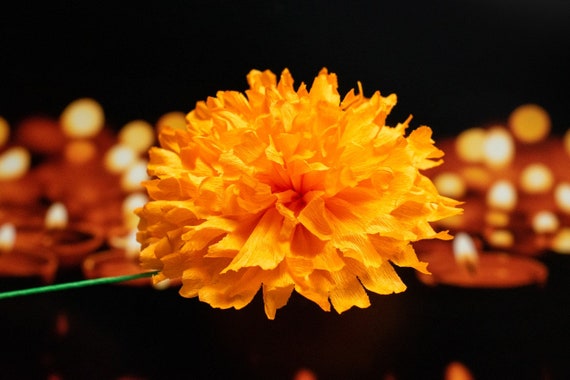The photograph showcases a striking yellowish-orange carnation flower standing proudly at the center, characterized by its multitude of delicate, rounded petals that start at the base and flourish upwards, creating a fluffy and pretty appearance. A small green stem can be seen holding the flower in place. The background is completely black, enhancing the contrast and making the flower stand out. Surrounding the central bloom, over 20 lit candles emit a soft, amber light, suggesting a serene or solemn ambiance. The candles are somewhat blurry, adding to the mystical feel, and might indicate a religious ceremony, a shrine for a tragic event, or a festive holiday. Overall, the image beautifully captures the interplay between the delicate flower and the gentle flicker of the candles against the dark backdrop, creating a visually captivating and emotionally evocative scene.